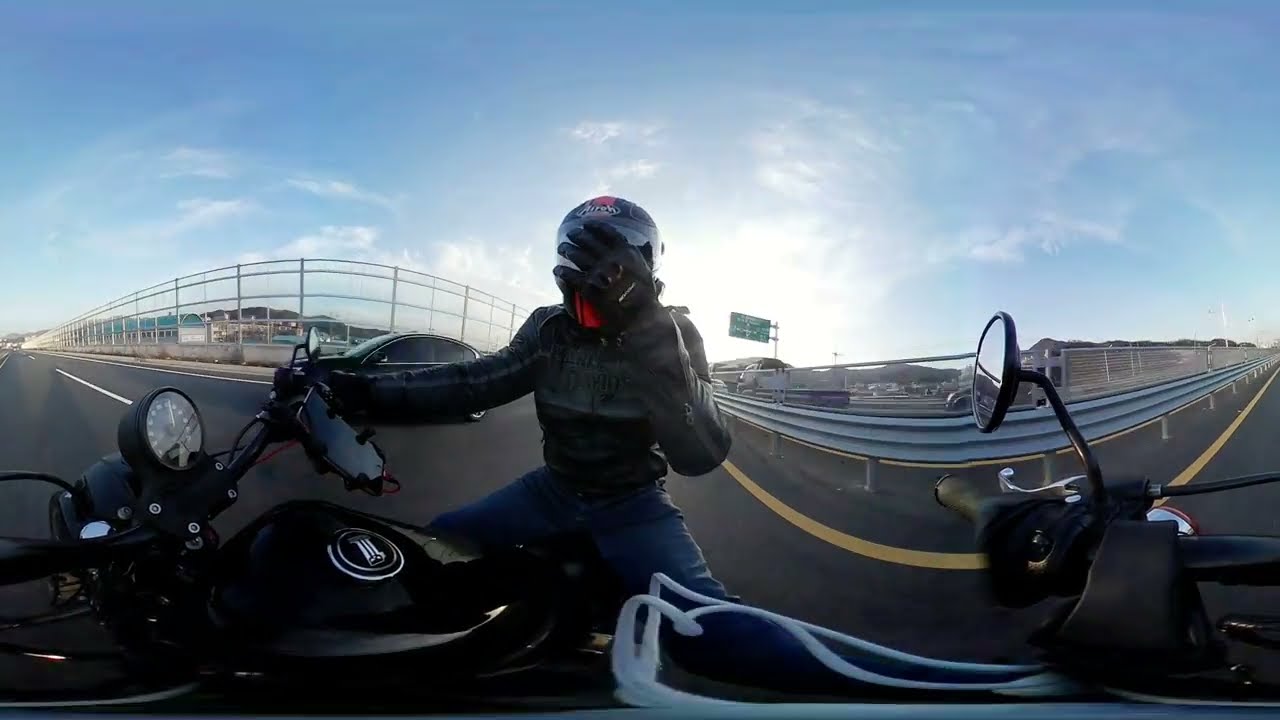In this dynamic image captured with a fisheye lens, we observe a motorcyclist, possibly male but indeterminate, on a large, black motorcycle, positioned prominently in the foreground. The cyclist is outfitted with a helmet, black gloves, a leather vest, jeans, and maintains a heavy-duty grip on the handlebars with his right arm, while his left arm is raised to his face, obscuring any facial features. A detailed array of instrumentation, including a speedometer or tachometer, is mounted on the handlebars.

The setting appears to be a highway on-ramp or off-ramp, characterized by black asphalt and yellow lane markings, with a tall, curving fence on the left, indicative of a possible overpass or bridge structure. In the lower right-hand portion of the image, the handlebar and rear-view mirror of a second motorcycle extend into view. Additionally, a black SUV can be seen riding parallel to the motorcyclist.

A prominent highway sign with green and white text looms over the cyclist’s left shoulder, typical of American roadways, suggesting navigation cues for upcoming exits. The landscape itself is relatively flat, extending into the distance under a low, blue sky with a sun near the horizon, hinting at a serene, late summer, spring, or fall day. The combination of these elements with the wide-angle distortion creates a surreal, immersive perspective, encapsulating both the immediate action and broader context of the road environment.